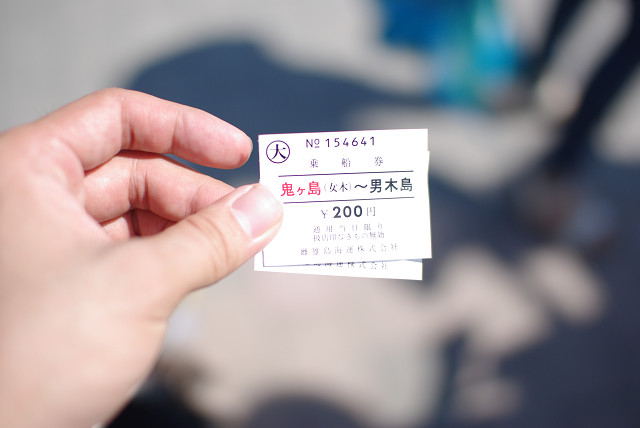The image shows a person with light-colored skin holding up two small white cards, one in front of the other, with their left hand. The hand’s thumb and middle finger are clearly visible gripping the cards. The front card prominently features a mix of red and black Asian characters, likely Chinese or Japanese, and the number "N0154641" at the top middle. Additionally, the number "200" is displayed in black at the bottom of the card. There is a circular logo containing an Asian character at the top left corner. The background of the image is out-of-focus, with hints of shadows and possibly a blue object, suggesting it was taken indoors in a room with white walls. The scene might depict the individual standing in line for an event.